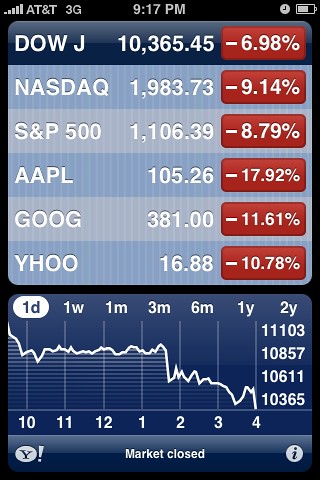The image is a screenshot from a mobile phone displaying stock market data, likely from an AT&T device, as indicated by the AT&T 3G label and the signal bars at the top. The time is 9:17 PM, with a battery icon and a small clock icon in the upper right corner. The display features six stock tickers: Dow Jones (10,365.45, -6.98%), NASDAQ (1,983.73, -9.14%), S&P 500 (1,106.39, -8.79%), AAPL (105.26, -17.92%), Google (GOOG, 381.00, -11.61%), and Yahoo (YHOO, 16.88, -10.78%). 

All stocks are showing significant declines, with percentages in red against a white font. Beneath these rows, a one-day line graph is highlighted, illustrating a pronounced downward trend from 10:00 AM to 4:00 PM. The graph is accompanied by numbers on the right, tracking the fluctuation of stock values throughout the day. The bottom part of the screenshot lists time increments from 10:00 to 4:00, with the YHOO logo and the words "MARKET CLOSED" centered below. There's also an 'i' inside a circle in the lower right corner, suggesting an information link. The screenshot predominantly features dark and light blue colors, with alternating light blue rows for each stock listing.